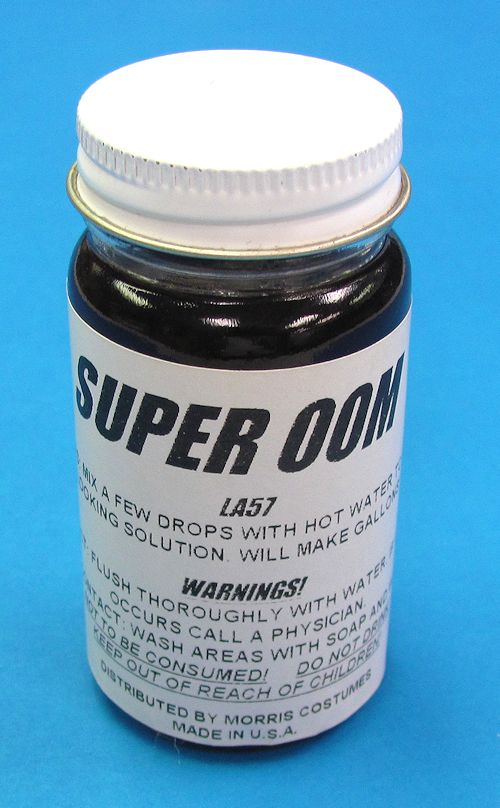This is a detailed photograph of a small glass bottle containing a black liquid, set against a solid blue background. The bottle features a white twist cap adorned with a gold or brass-colored rim. A prominent white label with bold black text covers much of the glass surface. Due to the curvature of the bottle, some text is partially obscured, but the following details are clear:

At the top of the label, the text reads "Super OOM" in a large font, followed by "LA57" in a smaller font. Below this, the instructions advise mixing a few drops with hot water, noting that a small amount of the solution will make gallons. Further down, the label includes various warnings such as "Flush thoroughly with water," "If a reaction occurs, call a physician," "Wash areas with soap," "Not to be consumed," "Do not drink," and "Keep out of reach of children." The bottle is distributed by Morris Costumes and is made in the USA.